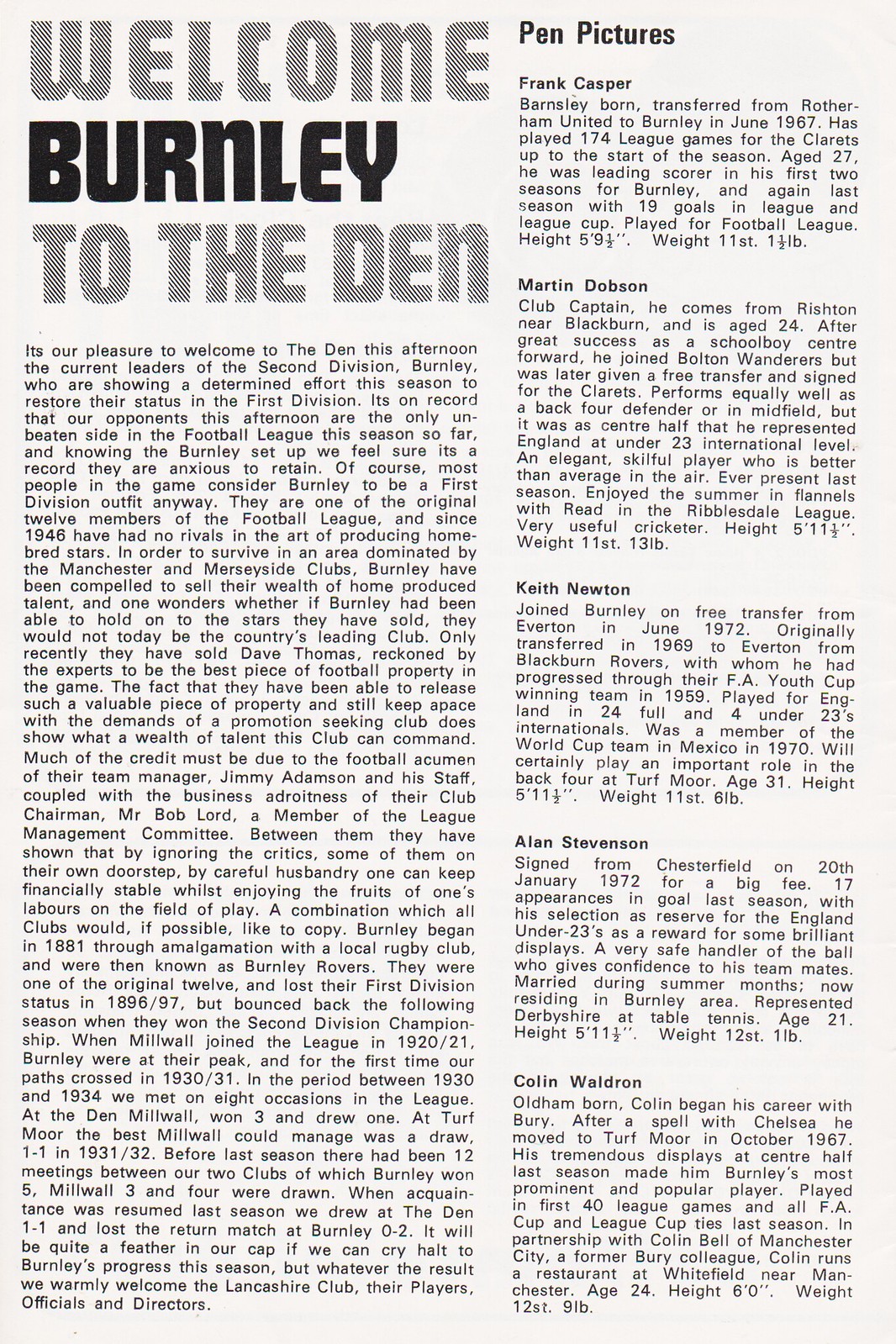The image is a vertically aligned, rectangular sheet of aged, off-white paper, resembling a page from a sports magazine or program. Dominating the top of the page are three lines of large, block letters, stating "WELCOME BURNLEY TO THE DEN" with 'Welcome' and 'To the Den' in gray, and 'Burnley' in black. Beneath this heading, on the left side, is a long, justified paragraph in black text, which celebrates Burnley's current standing as the unbeaten leaders of the 2nd Division and their efforts to return to the 1st Division. On the right side, under the bold heading "PEN PICTURES," are several sections, each titled with the names of football players such as Frank Casper, Martin Dobson, Keith Newton, Alan Stevenson, and Colin Waldron. Each name is followed by a justified paragraph providing details about the player. The text fills almost the entire page, with the colors mainly comprising off-white, black, and gray.